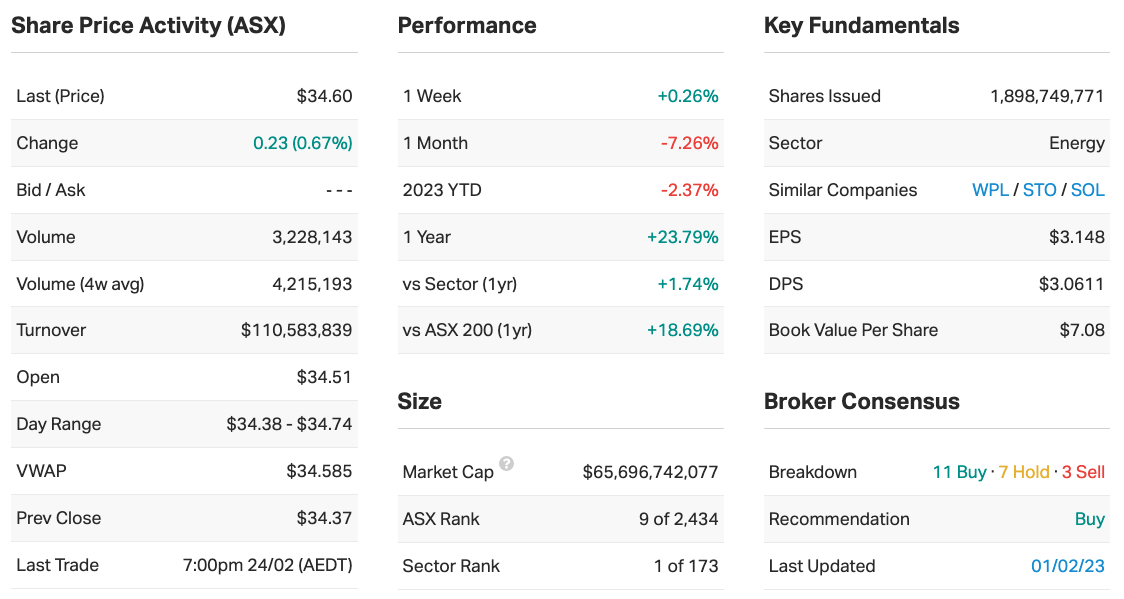Screenshot of Stock Performance on ASX Platform

The screenshot showcases detailed stock performance metrics on a white background, organized into three primary columns. The first column on the left, titled "Share Price Activity (ASX)," presents critical stock data including:

- Last Price
- Change
- Bid
- Ask
- Volume
- Turnover
- Open
- Day Range
- Previous Quote
- Last Trade

With all values listed in black except for the "Change," which is highlighted in green indicating an increase of 0.23 cents or 67.67%.

The second column, divided into two sections, is titled "Performance." It breaks down stock performance over varying timeframes: 

- One Week, showing a gain of 0.26% (green)
- One Month, showing a loss of 7% (red)
- Year to Date
- One Year

Below this section, there is an additional category labeled "Size."

The third column, also subdivided, is dedicated to "Key Fundamentals" and "Broker Consensus." In the "Key Fundamentals" section, similar companies such as WPL, STO, and SOL are listed, possibly indicating clickable links. In "Broker Consensus," the stock recommendations are color-coded:

- 11 Buy (green)
- 7 Hold (yellow)
- 3 Sell (red)

The timestamp or date is notably in blue, adding a unique touch to the color palette.

This structured layout provides a comprehensive view of the stock's current status and historical performance, making it a useful snapshot for investors.